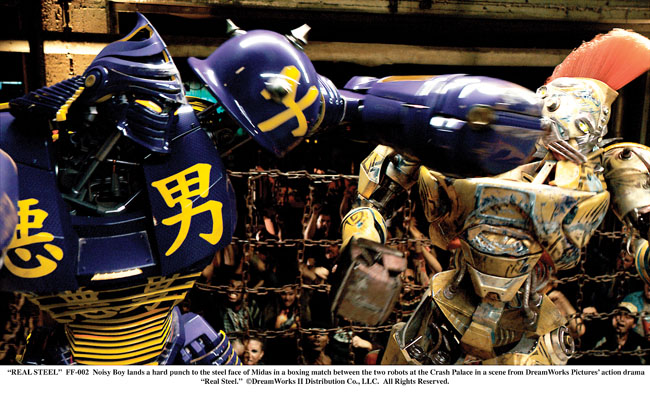This detailed photograph, likely a still from the movie "Real Steel," depicts an intense battle between two humanoid robots in an arena setting. The robot on the left is predominantly blue with yellow accents, including yellow eyes and Japanese characters on its chest. It is captured mid-punch, striking its opponent with its left fist. The robot on the right, styled with a distinctive orange mohawk, is primarily yellow with significant wear revealing underlying steel, giving it a bluish and silver appearance. Behind them, chains suggest they are fighting on a stage, with a crowd of humans visible in the background, seemingly cheering on the spectacle. The bottom of the image features text that reads "Real Steel," alongside other descriptive text.